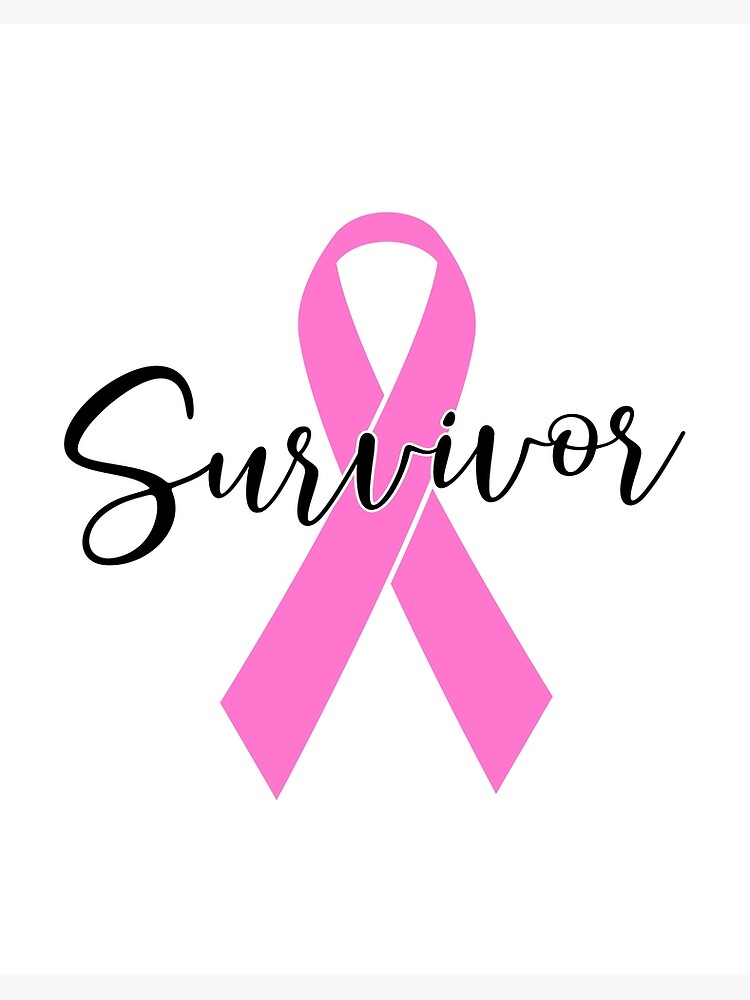Description: The image prominently features a pink cancer awareness ribbon, symbolizing breast cancer awareness. The ribbon is centrally located and neatly looped against a pristine white background. Across the midsection of the ribbon is the word "Survivor," elegantly scripted in black cursive letters. The overall composition is simple yet powerful, with no additional objects or text, allowing the ribbon and the word "Survivor" to convey their message of strength and hope unambiguously. The image is brightly lit, ensuring high clarity and a clean, focused portrayal of the ribbon and text.